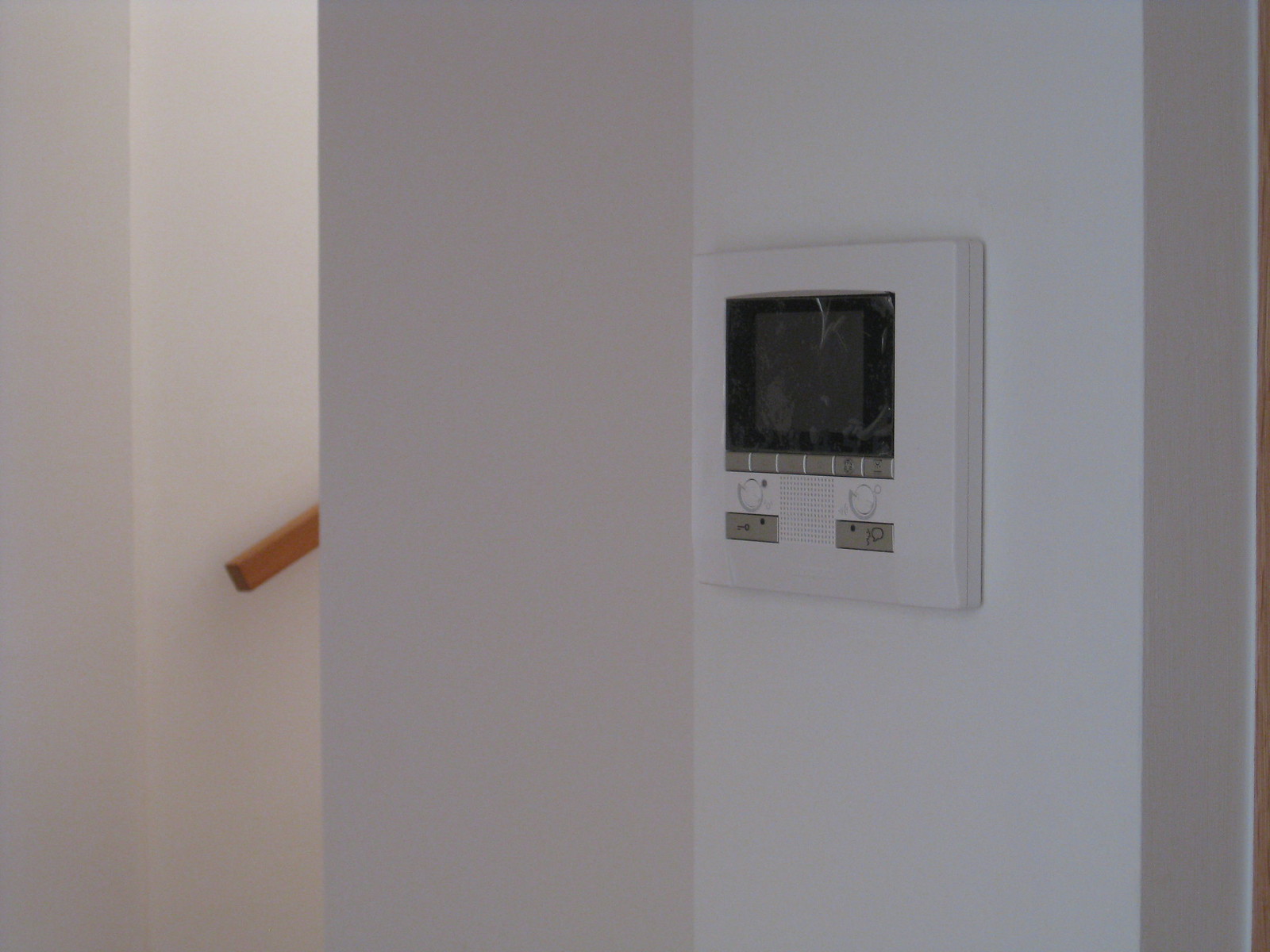In the image, we see a section of a completely white house interior featuring an alarm system mounted on one of the walls. The background reveals portions of other white walls, hinting at the expansive nature of the space. Towards the left side of the picture, a hand railing made of plain brown wood indicates the presence of a staircase leading downward, though the stairs themselves are not visible. This hand railing is illuminated by some natural light, suggesting an open staircase hallway.

The focal point of the image is the alarm system, a basic white box prominently featured against the angled wall. The device sports a black screen inset within a gray frame, still protected by its original plastic covering. Below the screen, there are six indistinct buttons, further supported by a functional layout that includes two knobs and a key mechanism. Adjacent to one of the knobs, there's what appears to be a voice box. The lower section of the device is somewhat obscured, but it likely contains additional components related to its alarm functionality or possible intercom features. The detailed arrangement of buttons, knobs, and the voice box supports the identification of this unit as an alarm system rather than an air conditioning control panel.